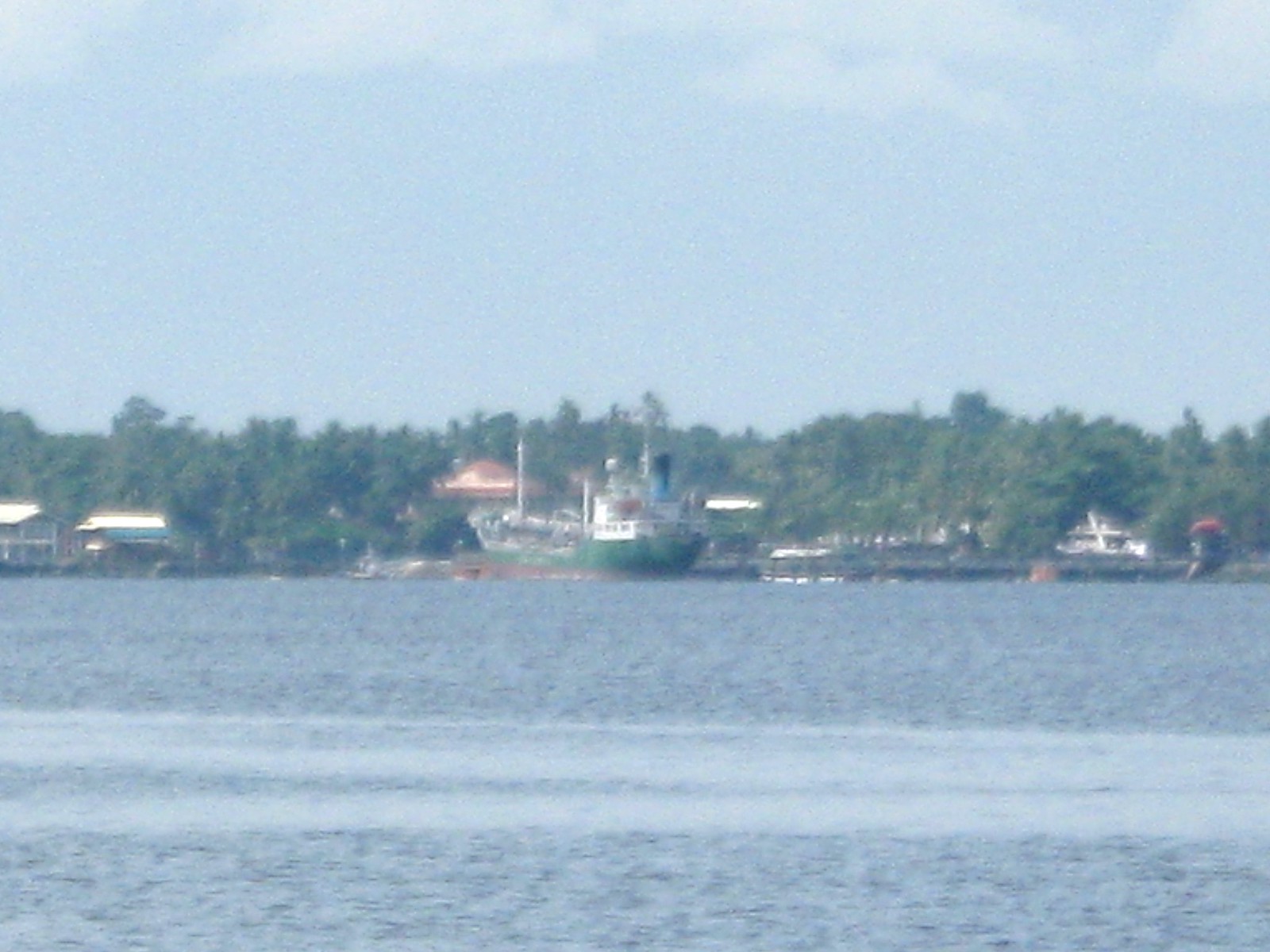The photograph is a rectangular, out-of-focus image that seems to have been taken from a boat or along a shoreline, featuring a large body of calm water that is somewhat disturbed where a boat likely recently passed through. In the center of the picture, there is a noticeable green and white boat, resembling a tugboat, with additional smaller boats flanking it. The background is characterized by a significant tree line that suggests a wooded area or forest. The sky above is blue, dotted with fluffy white clouds. Along the distant shoreline, there are several docks and smaller buildings, including a pier and structures with roofs in white and brownish colors. The overall color palette includes various shades of blue, green, red, brown, and tan.